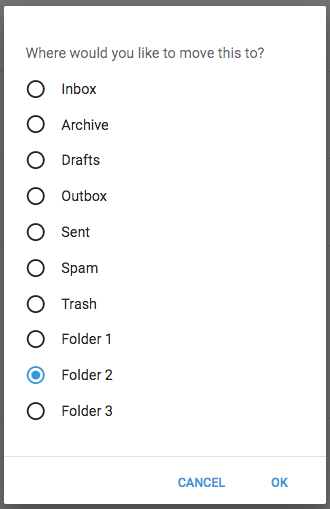The screenshot depicts a user interface window with a prompt asking, "Where would you like to move this to?" Various circular icons representing different folders are available for selection, each labeled respectively: Inbox, Archive, Drafts, Outbox, Sent, Spam, Trash, Folder 1, Folder 2, and Folder 3. Notably, Folder 2 is highlighted in blue, indicating the current selection. Below the folder options, there is a horizontal gray line, followed by two buttons on a white background labeled "OK" and "Cancel." Surrounding the elements in the screenshot are both a red and a black border. The image shows a straightforward decision-making process, where the user can confirm the choice by clicking "OK" or change their decision by pressing "Cancel." The interface is minimalistic, with no additional text, images, or options provided beyond those described.